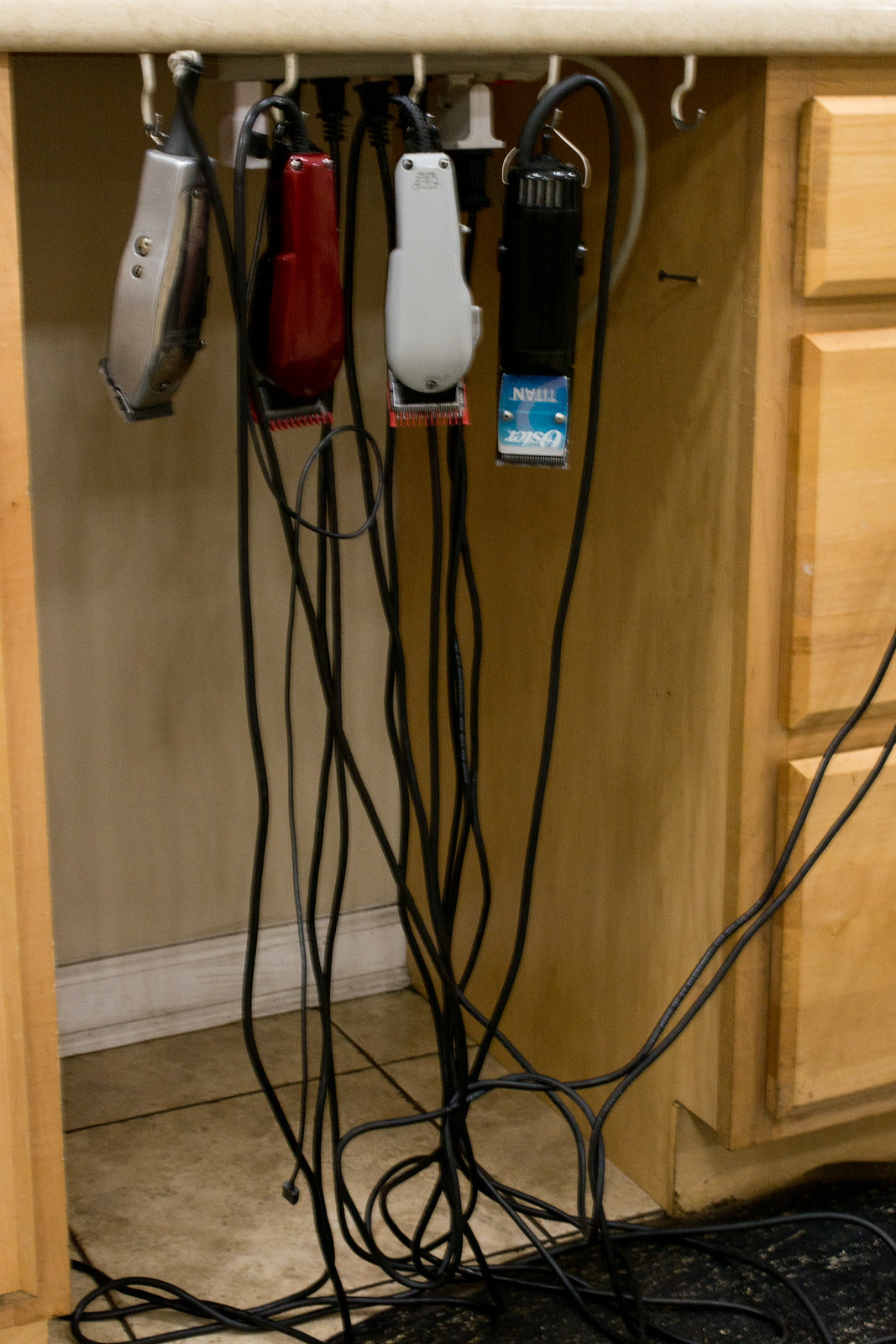The photograph showcases a highly detailed barber station set against a tan-colored wall with a white baseboard. The station features a wooden cabinet with a marble top, partially obscured, and a distinctive black rubber mat placed in front of it on a brownish-beige tiled floor. Prominently, four hair clippers of different colors—silver, red, black, and white—hang from white hooks mounted under the cabinet. These clippers are connected to a messy tangle of cords that trail out of the frame of the image. The detailed textures and colors of both the clippers and their cords create a visually intricate scene, complemented by another glimpse of brown cabinetry to the left and possibly drawers or additional shelves on the right.